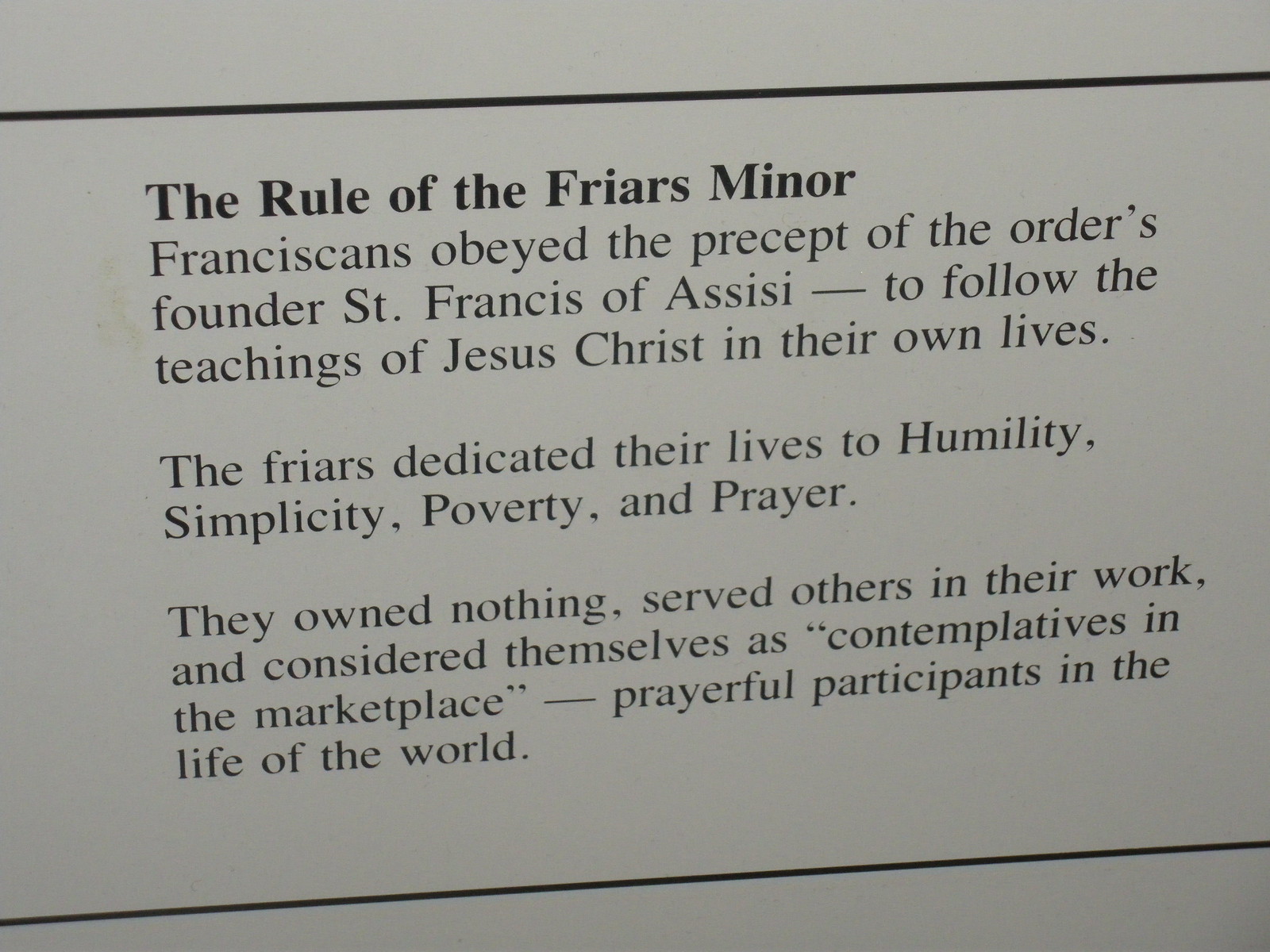This is a black-and-white photograph depicting what appears to be a printed page, possibly from a book. At the top, below a horizontal black line, it reads, "The Rule of the Friars Minor." Below this headline, three small paragraphs describe the principles followed by the Franciscans. The text states that Franciscans obeyed the precepts of their Order's founder, Saint Francis of Assisi, aiming to emulate the teachings of Jesus Christ in their lives. The friars, also referred to as Frères Minor, dedicated themselves to humility, simplicity, poverty, and prayer. They owned nothing, served others through their work, and saw themselves as "contemplatives in the marketplace," being prayerful participants in the life of the world.